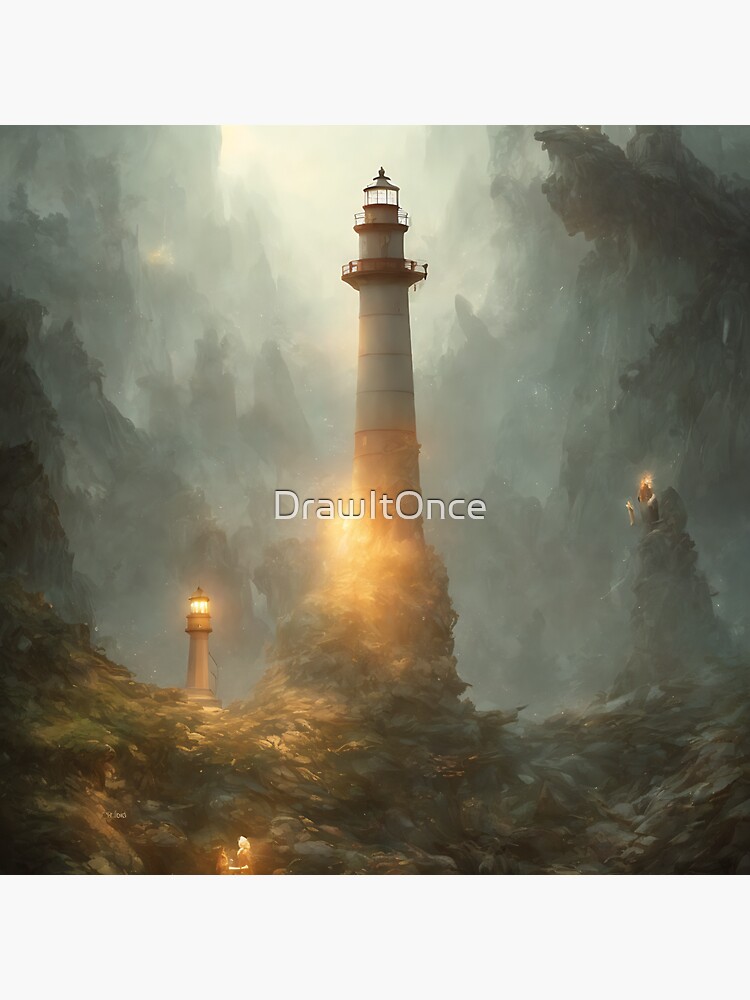This dramatic, dark, and misty painting depicts a fantasy landscape dominated by three lighthouses set within a steep, rocky valley. The central figure is a tall white lighthouse, prominently positioned on a towering rocky outcropping, illuminated at the top with circular lit windows and red railings. This main lighthouse, stark and bright against the dark background, has the phrase "DRAWIT" spelled out in bold white lettering across its center. To the lower left of it stands a smaller yet similarly shaped lighthouse, while another light source emerges from a rocky outcropping to the right, emanating light but adding ambiguity to whether it is a lighthouse or another type of structure. The surrounding valley is enveloped in a thick white mist, adding an eerie, otherworldly atmosphere to the scene.